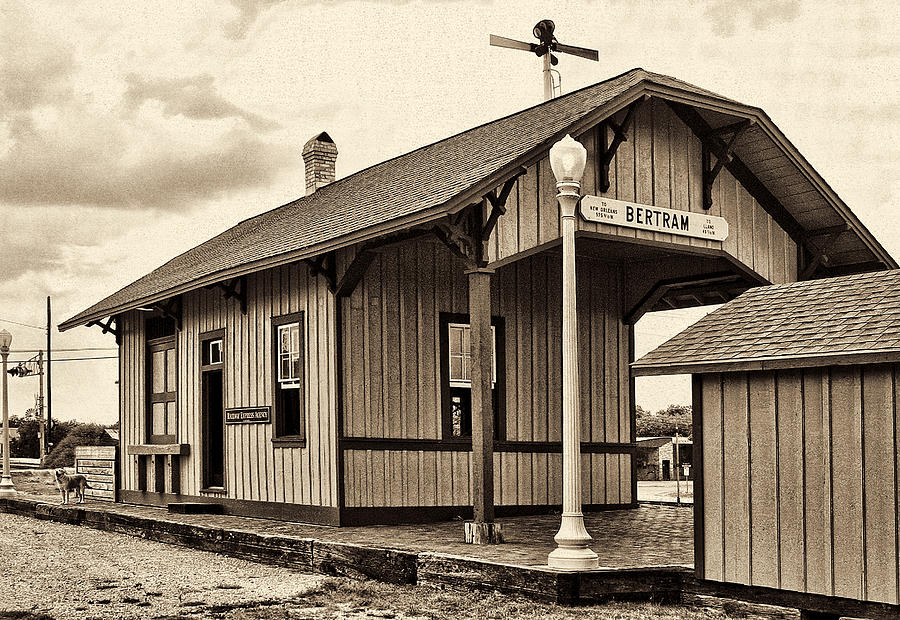The image depicts a small, rural, black and white railway station named "Bertram." The photo has a grainy, vintage texture, suggesting it is either an old or retro image. The station features a tiled roof and an overhang where people can take shelter from the rain. The exterior is composed of light-colored wooden panels. Adjacent to the building is a lamppost with an old street sign attached. The scene includes a smaller shed-like building, presumably used for storage, with a couple of open windows and a door with another closed window. The sky is overcast and cloudy, adding to the melancholic and deserted feel of the station. A small dog sits on the platform stoop in front of the main door, enhancing the rustic and abandoned atmosphere.